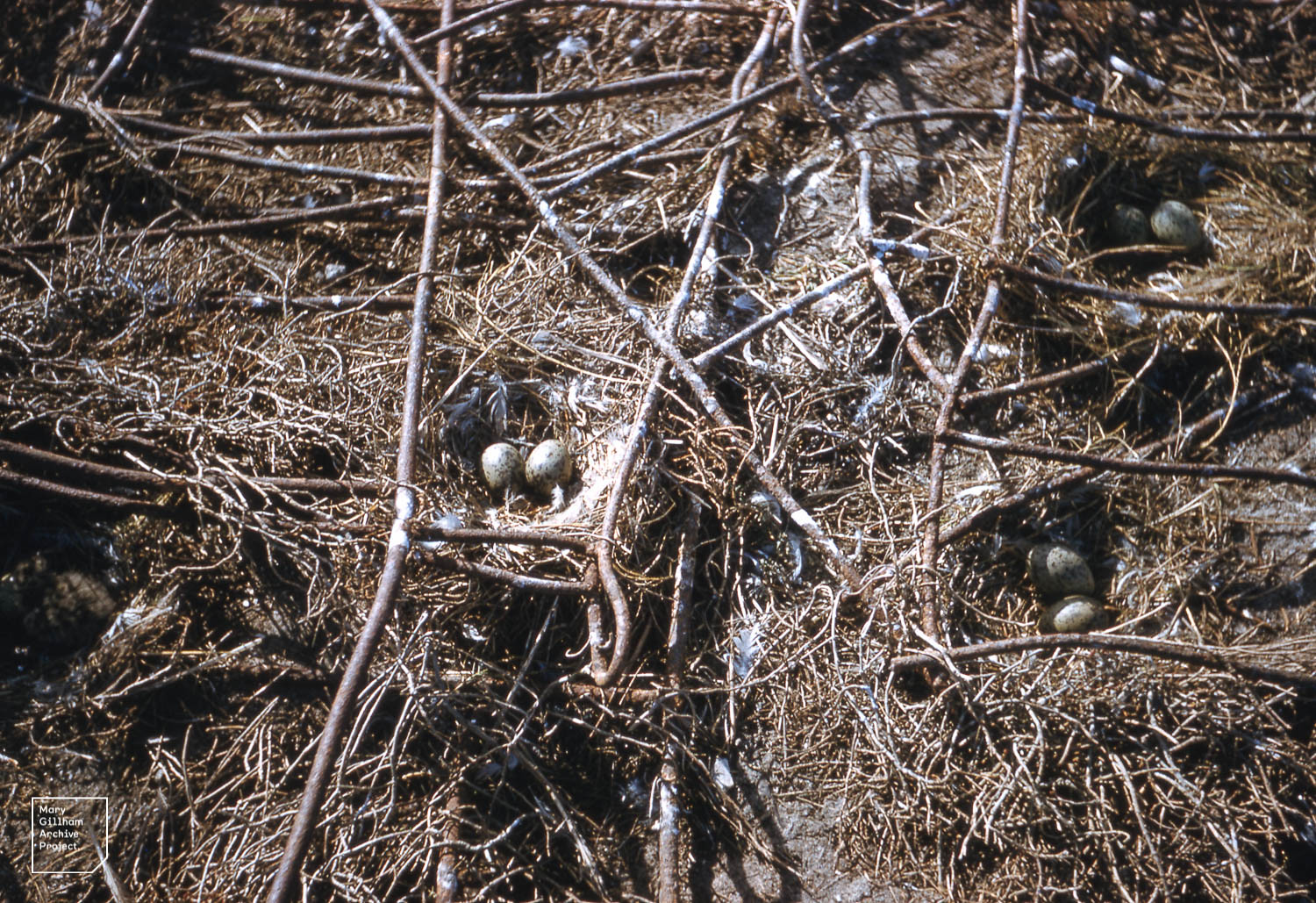The image shows a carefully constructed grid on the ground composed of twigs, branches, and brush, likely arranged by human hands. Within this grid are three bird nests, each containing two brown, speckled eggs, identifiable as killdeer eggs. The nests sit on a bed of gray and yellowish nesting material, amidst a mix of dead spruce and pine needles. The grid pattern is formed by overlapping sticks in a rudimentary square arrangement, providing structure to the nests. Scattered white killdeer feathers hint at the nesting birds' identity, although no animals are present in the scene. In the lower right-hand corner, the text "Mary Gilliam Archive Project" is visible, marking the origins of this detailed and serene nature snapshot.